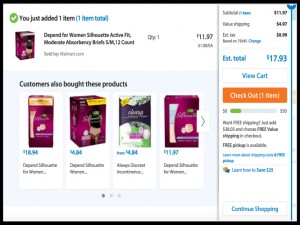Screenshot Description: The image is a small screenshot of a checkout page from an online shopping site. The page prominently features a section where a user has added an item to their cart: "Depend for Women Silhouette Active" — a product that appears to be designed for women and possibly related to hygiene products like tampons. The text is very small and hard to read clearly. 

On the right pane, there's a detailed breakdown of the estimated total cost, including item subtotal and taxes, amounting to $17.93. There are two prominent buttons for proceeding: a "View Cart" button and a notably orange "Checkout" button, contrasting against the white background. The interface has a user-friendly layout similar to Amazon's, with associated "Customers also bought" recommendations featuring similar products, many of which are packaged in purple boxes. Despite some text being too small to decipher, the overall design aims to facilitate an efficient shopping experience with options to continue shopping or finalize the purchase.